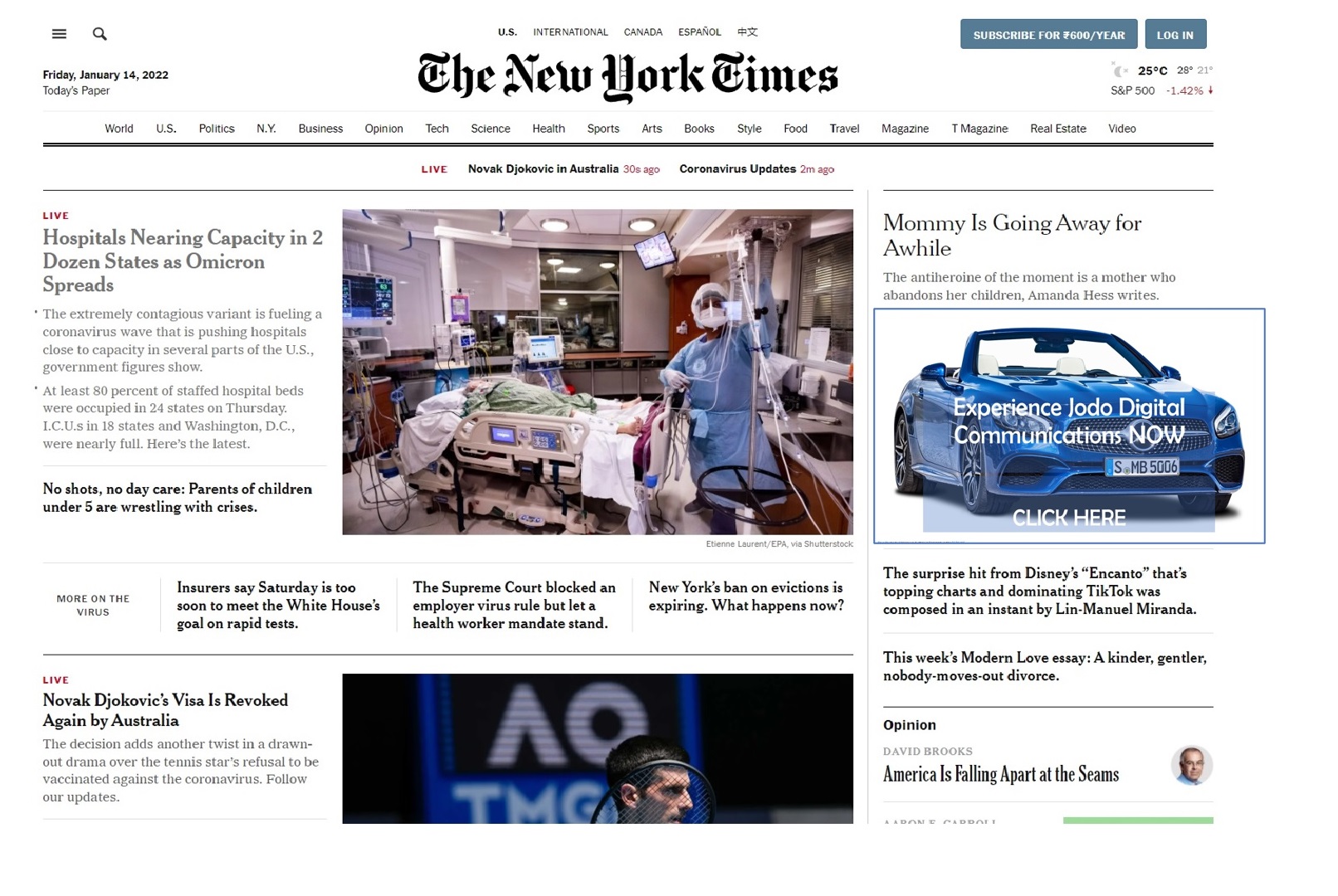A detailed screenshot from the New York Times website is shown. At the very top center, "The New York Times" is prominently displayed in an Old English black font. Above this title, five language selection tabs are visible, with the "U.S." tab on the far left currently selected. The adjacent tabs read "International," "Canada," "Español," and "中文" (Chinese). To the top left, the date is displayed as "Friday, January 14th, 2022," beneath which "Today's Paper" is written in a less bold font. 

On the top right, two dark turquoise boxes are present; the first box says "Subscribe for $600 per year," and to its right is a "Log In" option. Below this, the temperature is shown as 25 degrees Celsius, and the S&P 500 index is noted to be down by 1.42%. A black line separates these elements from the next section of navigation tabs. From left to right, the tabs read: World, U.S., Politics, N.Y., Business, Opinion, Tech, Science, Health, Sports, Arts, Books, Style, Food, Travel, Magazine, T Magazine, Real Estate, and Video. Beneath this, the website features multiple sections, indicating various content categories available for readers.